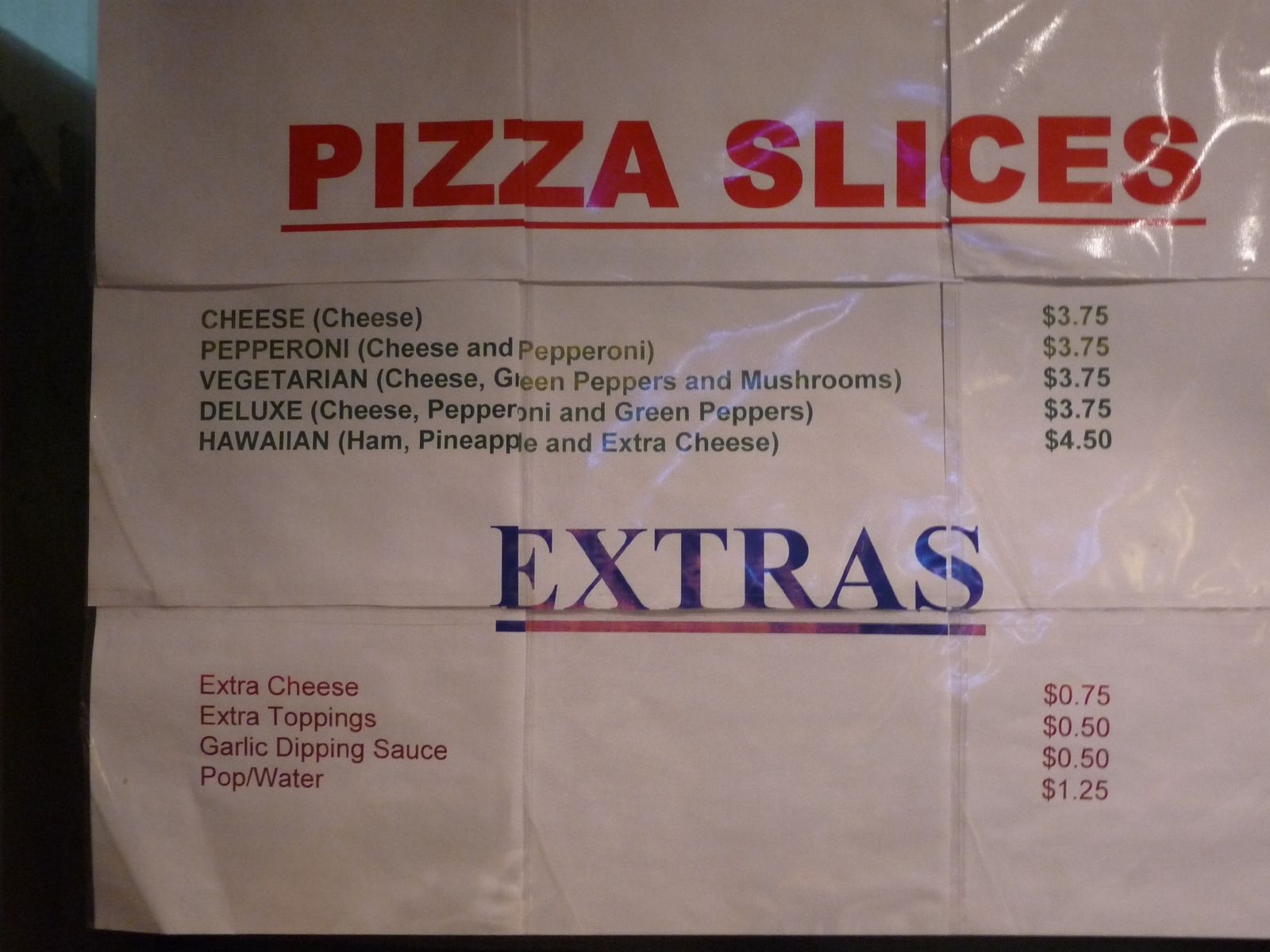The image showcases a simplistic, laminated menu consisting of three sheets of paper stacked and folded for durability. The top section prominently features the bold, uppercase title "PIZZA SLICES," with an underline for emphasis. Below, the middle sheet lists the types of available pizzas, with most priced at $3.75. Options include Cheese (just cheese), Pepperoni (cheese and pepperoni), Vegetarian (cheese, green peppers, and mushrooms), and Deluxe (cheese, pepperoni, and green peppers). The Hawaiian pizza, which includes ham, pineapple, and extra cheese, is priced slightly higher at $4.50.

The bottom section, titled in capitalized and underlined "EXTRAS" in purple, offers additional items: extra cheese for $0.75, extra toppings for $0.50, garlic dipping sauce for $0.50, and pop and water for $1.25. The straightforward, no-frills presentation suggests this menu belongs to a local hometown pizza joint.